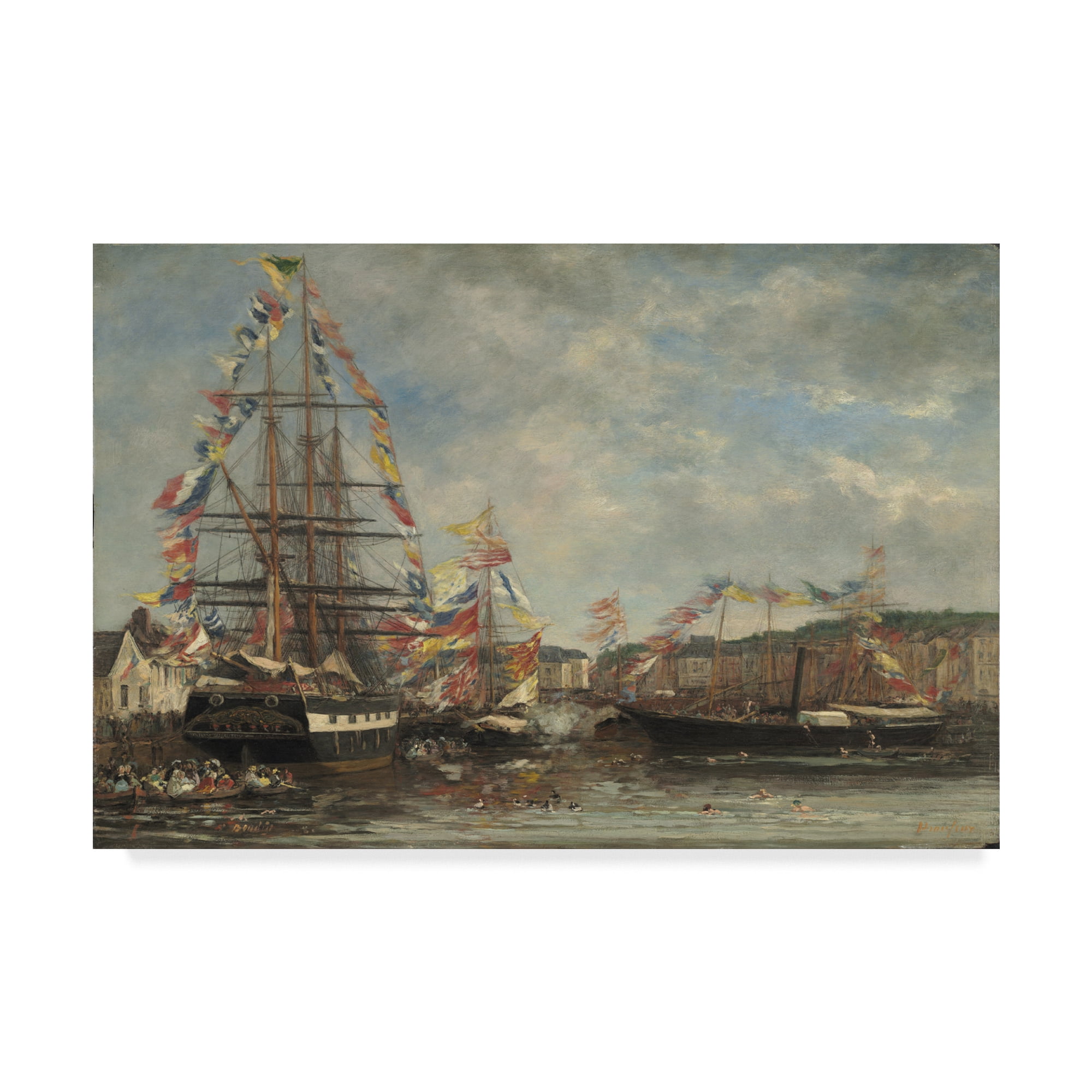This painting depicts a vibrant harbor scene under a blue sky filled with fluffy white and gray clouds. The foreground features three ships adorned with multicolored flags—predominantly red, white, yellow, and blue—draped across their mast and sail lines. The largest ship, positioned centrally, commands attention with its towering mast and intricate posts, almost reaching the top of the image. It faces forward, showcasing its black-and-white hull, and is festooned with flags reaching up its towering structure. 

To its right, a smaller ship mirrors the colorful display, with flags hanging around the top and rising mid-height up the larger ship's posts, and it is oriented towards the larger vessel as if in conversation. On the bottom right, the smallest ship, which also features the same vibrant flags, faces the larger ship. 

The water below the ships is dotted with activity: ducks float serenely, and there are small boats and rowboats full of people navigating the harbor. On the left, adjacent to the largest ship, figures are seen swimming, adding life to the scene. 

In the background, a picturesque small village or town rises around the dock, with stone townhomes and green hills completing the serene yet bustling landscape.